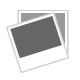The image depicts a red and gold circular object, which could be a decorative lid or the top of a short drum, laid upon a light-colored wooden surface. The object features a detailed design that includes a gold ring near the edge and a rope-like figure forming a cross or star shape drawn on its surface. It is situated against a white brick wall, suggesting the setting is an indoor corner of a building. The white brick wall appears to have been painted over darker bricks, contributing to the overall aesthetic of the scene. The black and red hat with a brim and a lid also contributes to the complex ambience of the image.